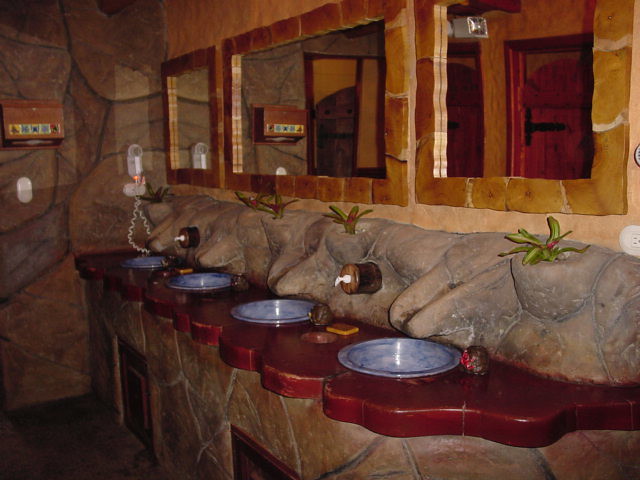This photograph captures a unique public bathroom designed with elaborate stone motifs, giving it an almost cave-like appearance. The walls are decorated with large, rust-brown stones interspersed with black mortar, contributing to an earthy, natural aesthetic. Running along the right side are four blue, marble-patterned sink basins set within a thick, wavy-edged, dark reddish-brown countertop that resembles polished rock. Above these sinks, three mirrors, each framed by tan stone bricks, reflect the room's interior. The mirrors are positioned such that two smaller mirrors flank a larger central one, aligning with the middle sinks. Along the countertop's length, built into the stone wall above, are soap dispensers, and to the left, a corded telephone can be seen. Additionally, there are green plants integrated into the design, with five areas behind the sinks featuring greenery and red flowers, enhancing the natural theme of the space. Notably, a white device, possibly a hand dryer, is mounted on the wall, adding a modern touch to the room's rustic charm.